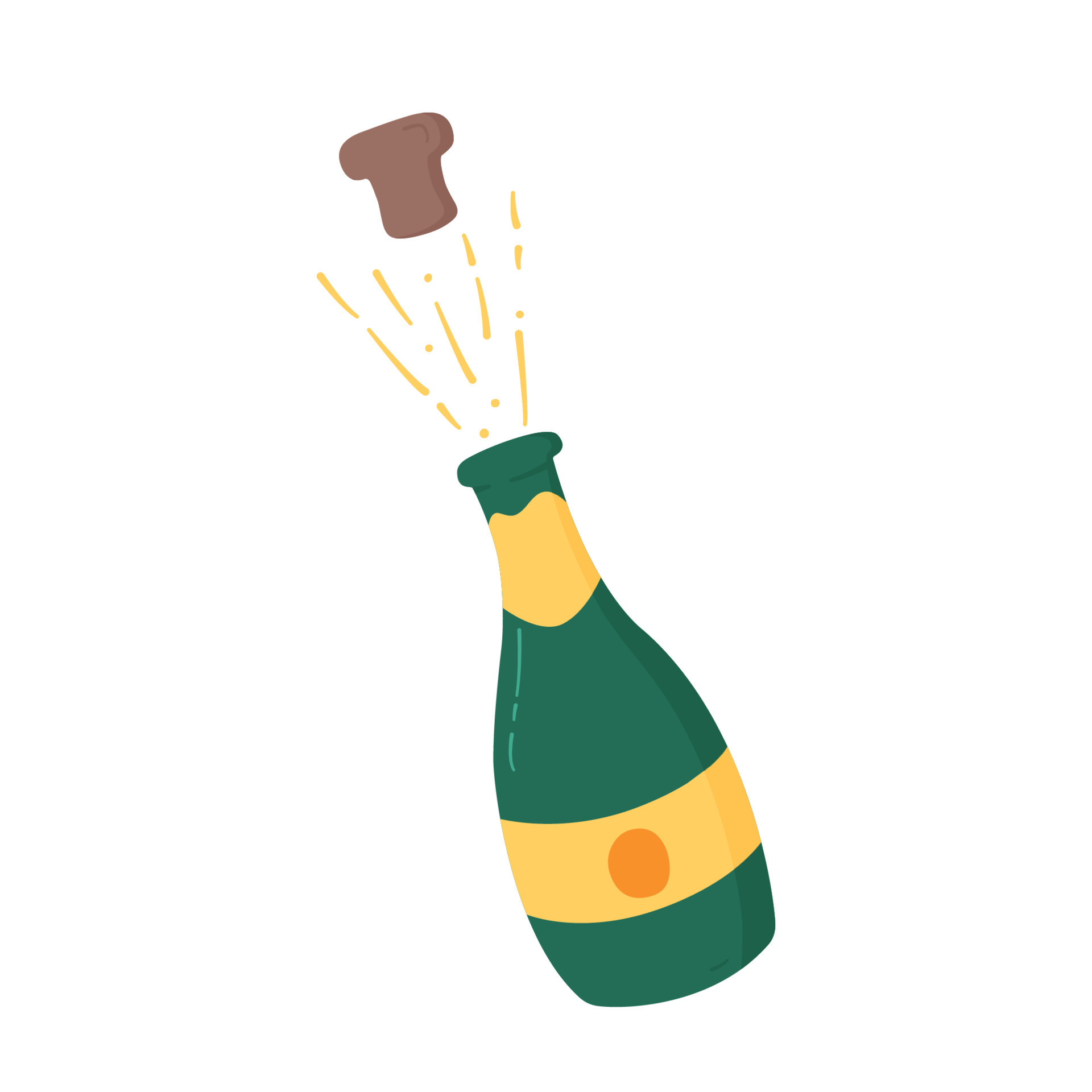This image is a cartoonish clip art of a celebratory champagne bottle on an infinite white background, commonly associated with events like New Year's, holidays, anniversaries, or birthdays. The green champagne bottle features a prominent yellow design at the neck, which is heart-shaped and wraps around to form a decorative label. The base of the bottle has a rectangular yellow label with an orange circle in the center. The bottle is angled slightly to the left at about 30 degrees. The cork, depicted in a dark tan color, has just popped out with force, angled towards the upper left corner. Yellow lines and spray marks emanate from the neck of the bottle, indicating the motion and energy of the popping cork. The overall image captures the festive moment of popping open a bottle of champagne with vibrant green, yellow, and orange hues against a stark white backdrop.